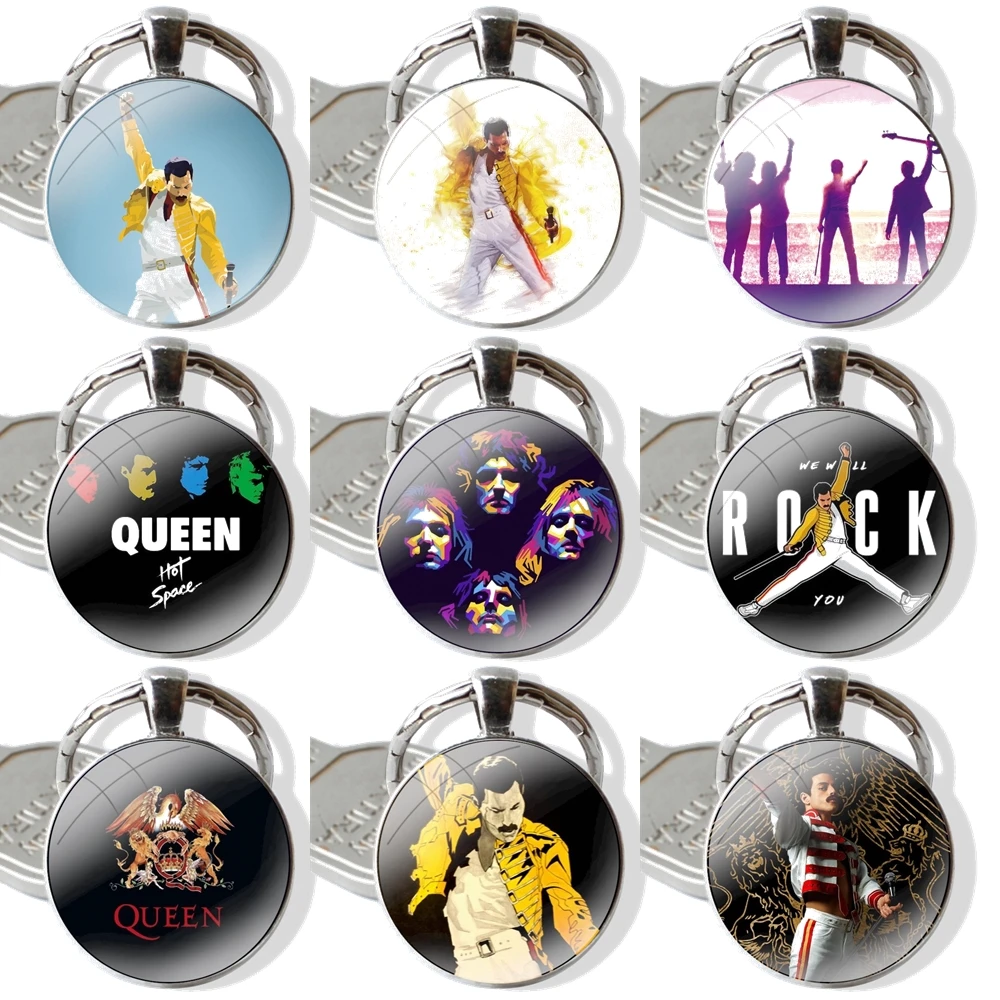The image showcases nine distinct keychains, arranged in three rows and three columns, each featuring a circular medallion front. These keychains are all dedicated to the iconic rock band Queen and its legendary frontman Freddie Mercury. 

From left to right, starting with the top row: 

1. The first keychain displays Freddie Mercury in one of his iconic poses, wearing a golden jacket against a blue background.
2. The second keychain features Freddie sporting a feathered jacket with a white background, enhanced by wispy designs. 
3. The third keychain depicts the back view of Queen's band members facing an ocean, with one holding a guitar aloft.

In the middle row from left to right:

4. The first keychain showcases the iconic "Bohemian Rhapsody" image of the four Queen members' faces in a shadowy collage, coupled with the text "Hot Space."
5. The second keychain presents the same four faces of Queen arranged in a diamond pattern.
6. The third keychain has a cartoon version of Freddie Mercury posing with the caption "We Will Rock You."

In the bottom row from left to right:

7. The first keychain displays Queen's official logo.
8. The second keychain shows a close-up of Freddie Mercury mid-performance.
9. The last keychain is a stylized image of Freddie with closed eyes, delivering a different type of performance pose.

The keychains have gray metallic backgrounds and glass circles with images, adding a collectible touch for any Queen fan.